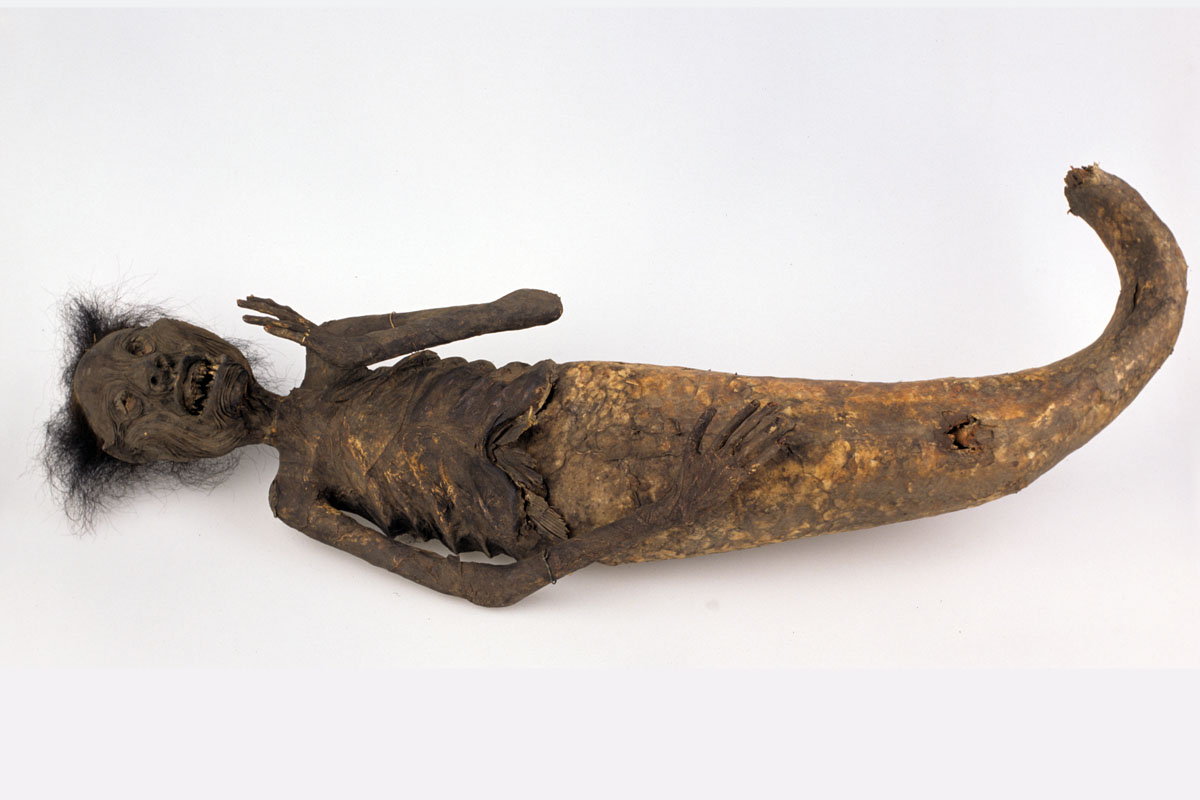The image features a dark brown, mummified corpse, centrally placed, with its head oriented to the left and a large tail extending to the right. The unique body structure resembles a mermaid or human-fish hybrid, with the upper body’s skeletal ribs prominently visible. The corpse’s left hand is raised, and its right arm is stretched downward, resting on the tail-like structure, which transitions from an orangish-tannish hue at the base to a thinner, curved end. The head displays patches of black hair, and an open mouth adds to the eerie effect. The background is a very light grey, enhancing the stark, grim appearance of the figure.